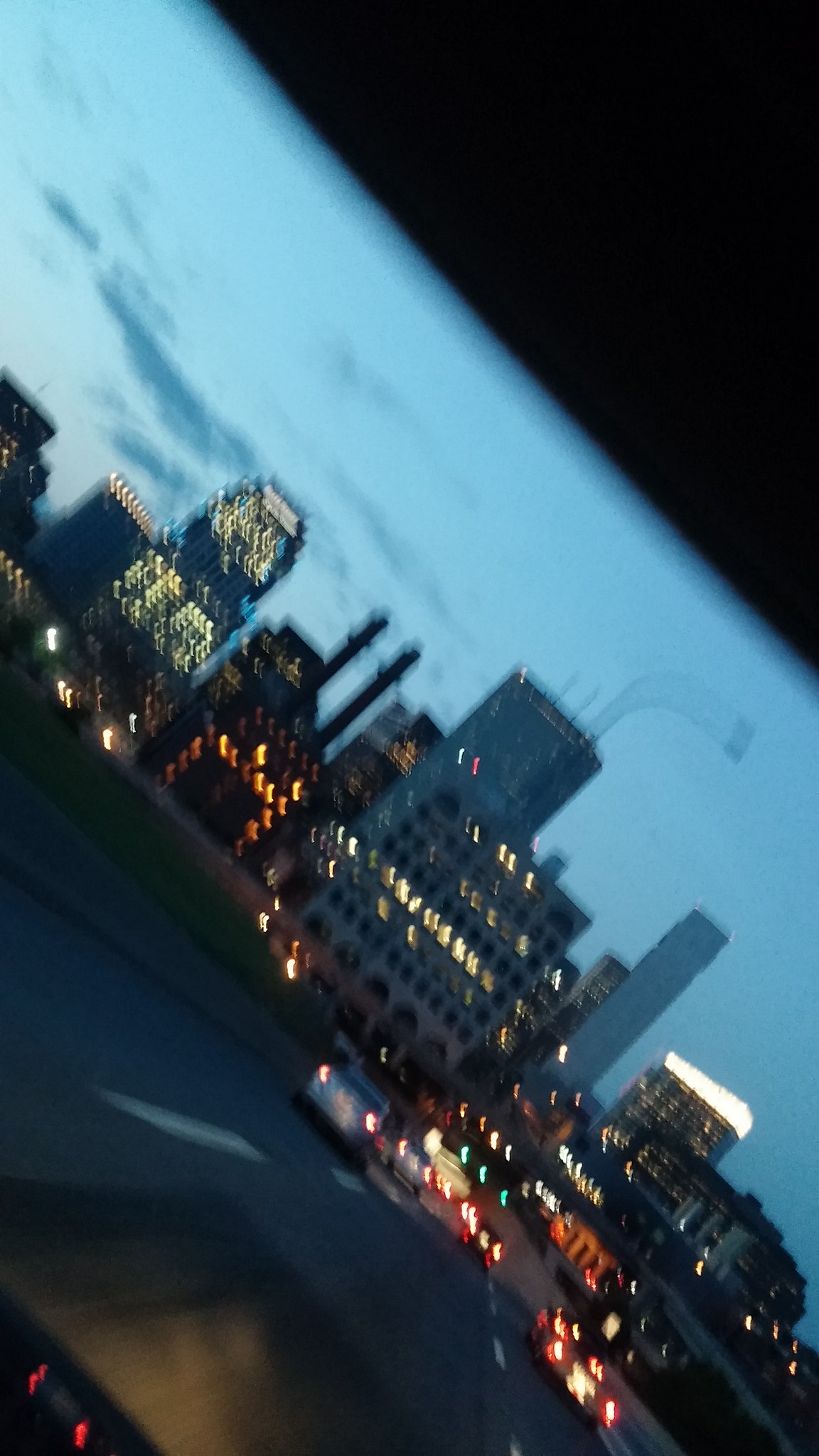The image is a blurry, dutch-angled photograph taken from inside a car, likely from the right-hand passenger side, showcasing a driver's point of view on a busy highway. The road, gray with intermittent white lines, is populated with seven cars, their brake lights aglow. The photo captures the vibrant cityscape ahead, featuring a mix of tall and short buildings of varying colors, including black and white skyscrapers with lit windows. Notably, there are two long pipes visible against a backdrop of a blue sky peppered with clouds. In the bottom left corner, the top of the dashboard is visible, showing two red lights. There's also a side rail and a small grassy area by the street, adding to the urban tapestry presented in the image.